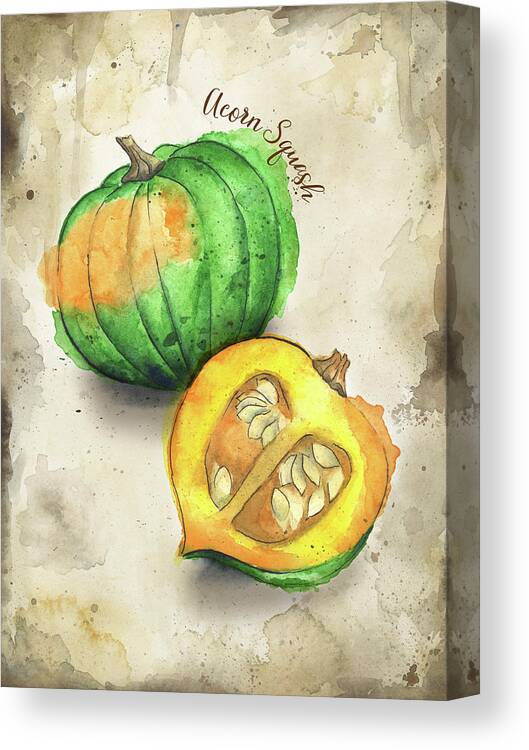The image showcases a watercolor painting on a small, worn canvas with a distressed, off-white background accented by gray and light brown splotches, giving it an aged appearance. Central to the painting are two acorn squashes. The first squash, depicted whole and primarily green with a small orange patch near the top, displays its stem and exterior. Adjacent to it, a second acorn squash lies cut in half, revealing its seeded core and vibrant yellow-orange flesh. Above the squashes, the text "acorn squash" is inscribed, identifying the subject matter of this detailed and textured artwork.